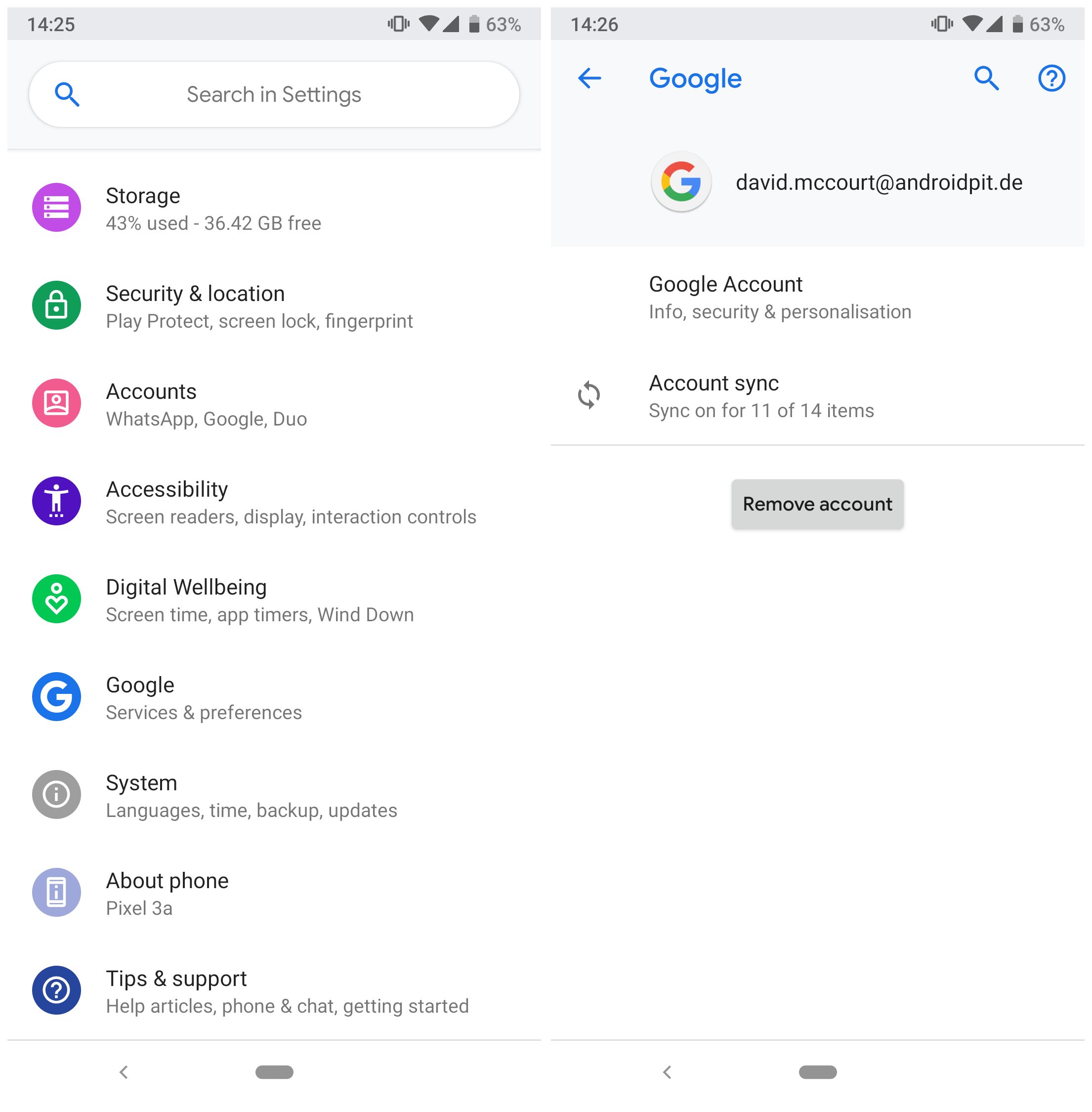The image consists of two side-by-side screenshots from a user's phone, each displaying various settings and options. 

- **Screenshot on the Left:**
  - **Time:** 14:25
  - **Status Indicators:** Vibrate mode active, full Wi-Fi signal, full cellular signal, 63% battery life
  - A search field labeled "Search in settings" is present, accompanied by a magnifying glass icon.
  - Below the search field, there are multiple setting options with colorful icons:
    - **Storage:** Displayed as a server stack inside a purple circle. It shows that 43% of the storage is used with 36.42 GB free.
    - **Security & Location:** Represented by a green circle with a lock icon. It lists features like Play Protect, screen lock, and fingerprint settings.
    - Other entries include **Accounts & Accessibility, Digital Well-being, Google, System, About Phone,** and **Tips & Support.**

- **Screenshot on the Right:**
  - **Time:** 14:26
  - **Status Indicators:** Identical to the left screenshot (Vibrate mode, full Wi-Fi, full cellular signal, 63% battery life)
  - At the top, there is a back arrow followed by "Google" in blue text, a magnifying glass, and a question mark in a circle.
  - The screenshot features a Google account area, showing the Google "G" inside a circle next to the username, david.mccourt at androidpit.de.
  - Beneath the username, it states "Google account info security and personalization."
  - There is a section labeled **Account Sync**, indicating that sync is on for 11 of 14 items, along with refresh arrows.
  - At the bottom, a gray button with black text reads "Remove account."

This detailed description captures the essential elements and options shown in the two side-by-side screenshots from the user's phone.